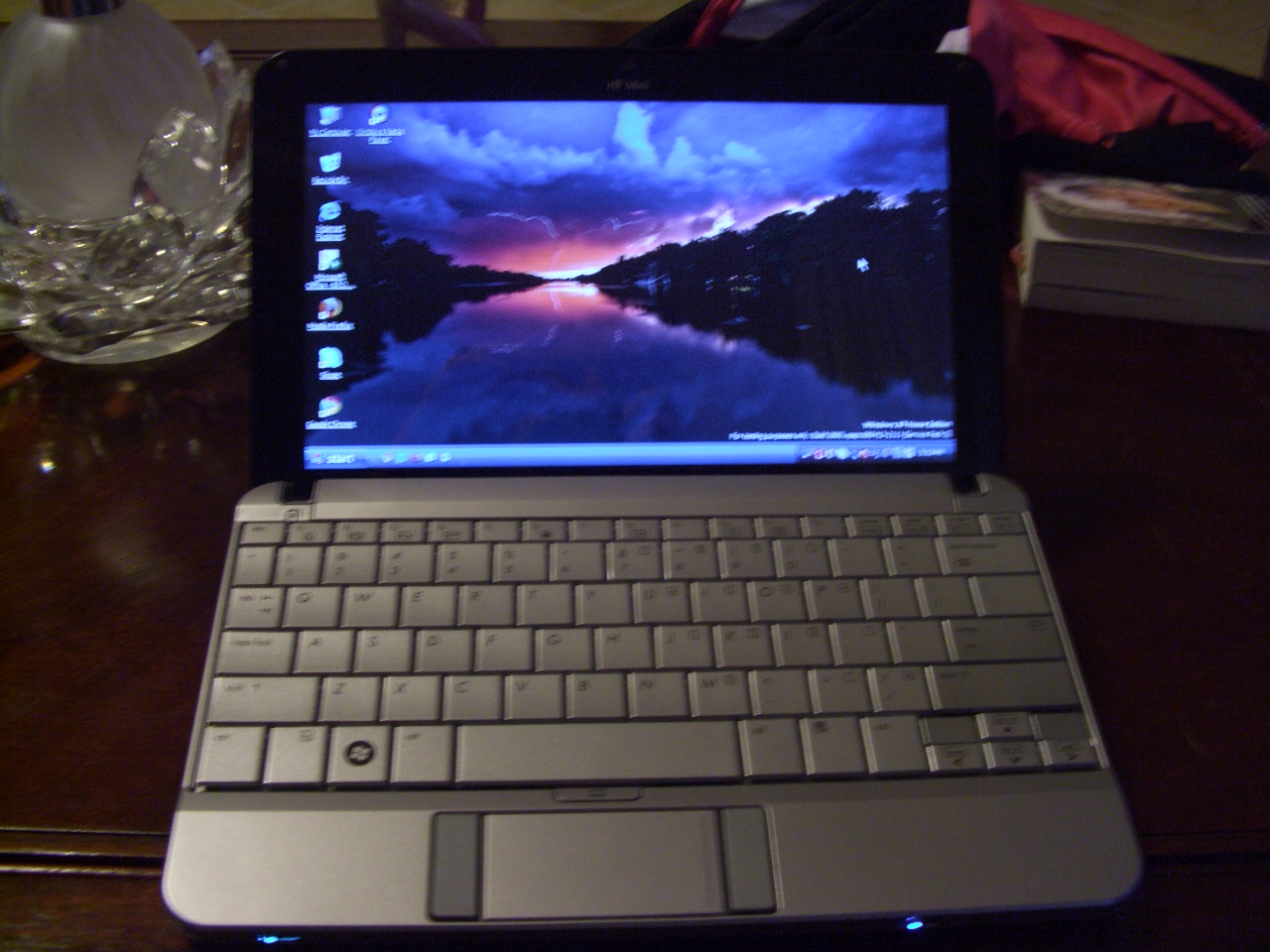The image depicts a silver laptop, possibly an HP, sitting on a brown wooden desk. To the left of the laptop, there is a crystal candle holder or glass vase. On the right side, a paperback book with a visible bookmark and a cover featuring a woman's face can be seen. Behind the book, there appears to be a red and black jacket, along with a pink clothing item, likely lingerie. The laptop is open with its screen extended, displaying a vivid screensaver. The screensaver features a dramatic sunset scene with sharply defined clouds, a vibrant fiery yellow sky blending into a purplish-blue hue, and a river flowing into the sunset. The picturesque landscape includes dark silhouettes of trees, possible homes with lights, and reflections on a lake.